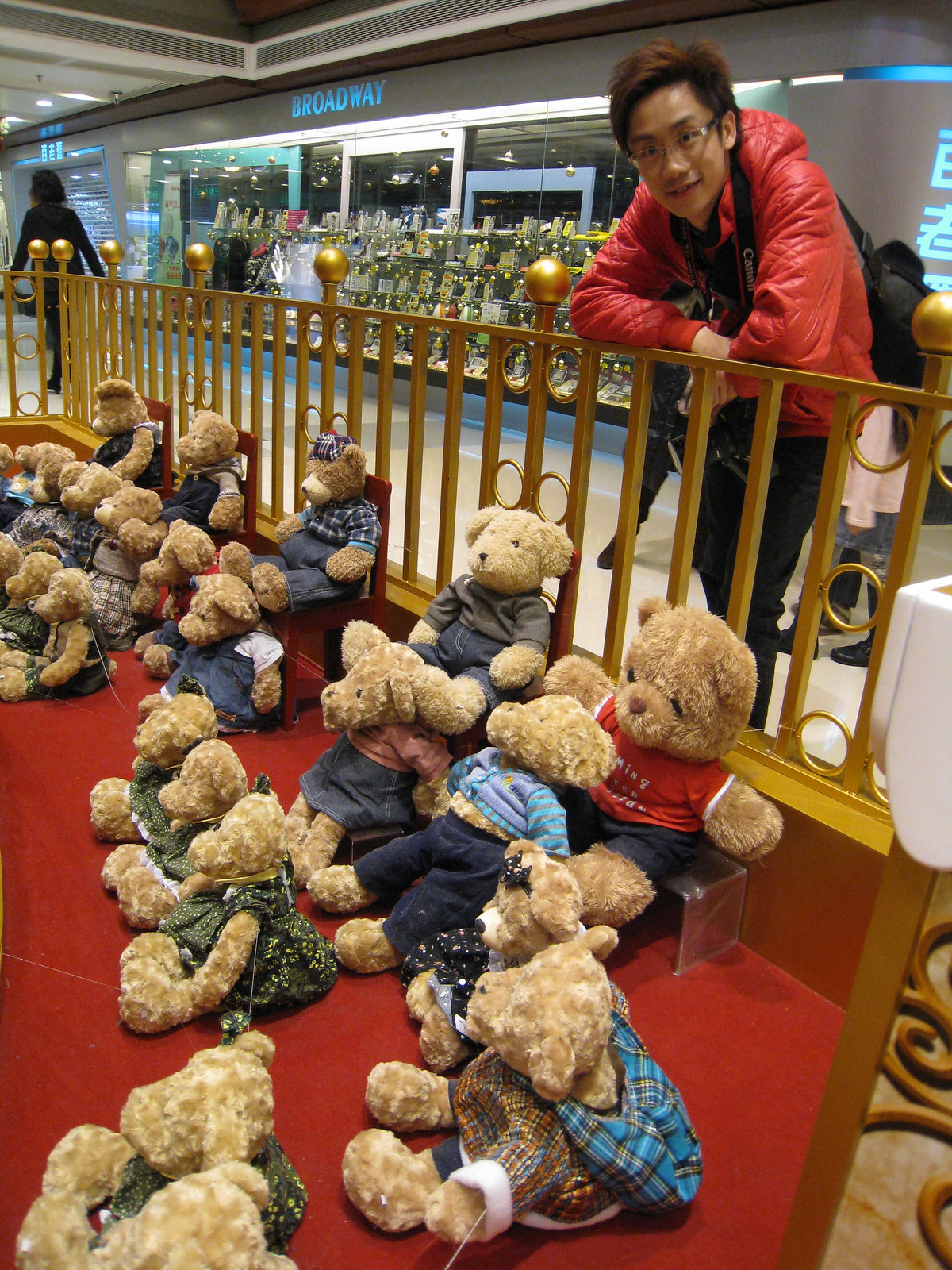This photograph, taken inside a mall, depicts a Build-A-Bear style exhibition centered in the walkway. A golden-colored fence with ornamental posts encloses the exhibit, which features a red carpet adorned with approximately two dozen brown teddy bears. The bears are dressed in various outfits, including shirts, jackets, pants, and dresses, in shades of blue, red, and green, and are arranged in groups of threes and fours, seated on both chairs and the floor. To the right of the display, an Asian man with glasses, brown hair, and a red puffer coat, wearing a black backpack and dark jeans, is leaning against the fence looking directly at the camera. In the background, the mall corridor extends with numerous stores displaying signs with Chinese lettering. Notably, a store named "Broadway" stands out with blue neon letters and has an array of glasses in the window. A woman dressed in black with black hair walks by on the left side of the image.